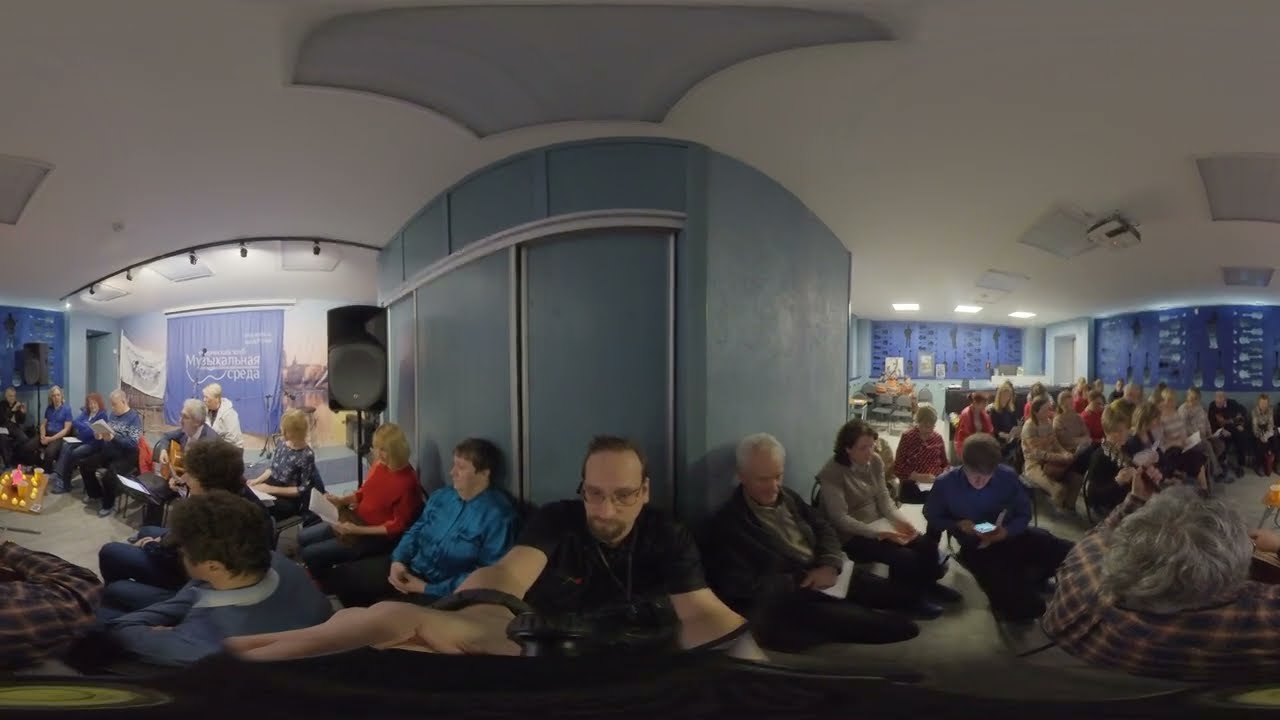The panoramic photograph captures a dimly lit, large waiting area or conference center with blue walls and a white ceiling. The room features a soft teal blue center wall and darker blue back walls. There are rows of dark black cushioned chairs occupied by middle-aged individuals, most of whom are holding papers or magazines, engaged in various activities such as staring into space or looking at their phones. A soft purple curtain with white lettering is visible on the left side, but the text is unreadable. The image also shows a person with a guitar and speakers, suggesting a musical performance. Another speaker and a table stand, possibly with flowers, are noted in the background. Overall, the scene is somewhat somber and quiet, with minimal lighting except for a few illuminated spots along the walls.